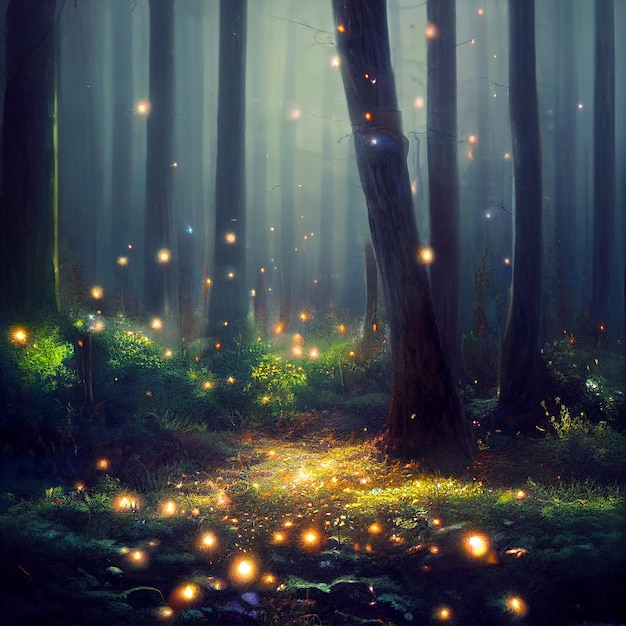This detailed illustration portrays a dark nocturnal forest bathed in an enchanting glow from numerous floating orbs of yellow light. The scene suggests a blend of nature and fantasy, possibly depicted through computer animation. Tall trees dominate the image, their silhouettes towering upwards with most branches obscured, emphasizing their immense heights. The forest ground is rich with vibrant green grass, moss, and dense underbrush. Interspersed among the vegetation are a few scattered rocks. Mystical lights, resembling fireflies or magical luminescent orbs, hover throughout the scene, some high up among the tree trunks while others nestle near the base, casting a gentle, magical illumination that reveals the textures and greenery of the landscape. A subtle, soft blue mist lingers in the background, enhancing the tranquil and mysterious atmosphere of this forest night.